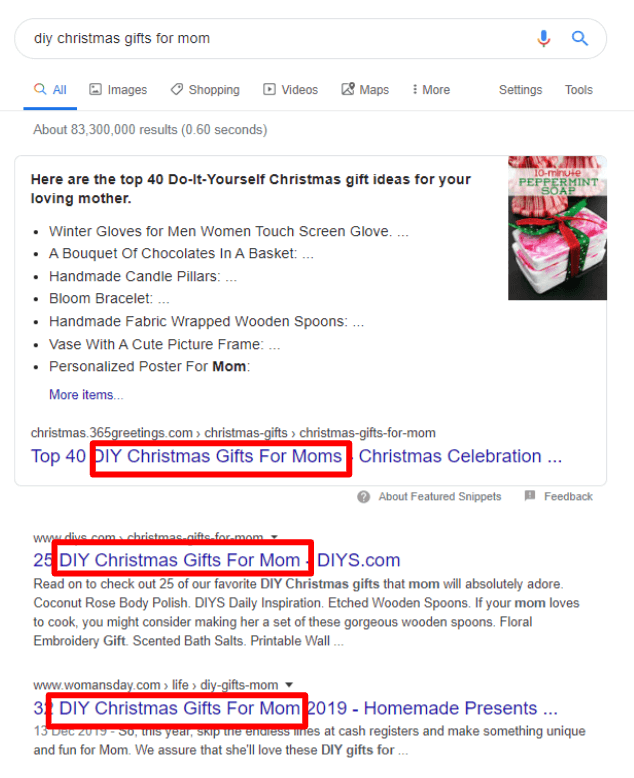A screenshot of a Google search for "DIY Christmas gifts for mom" on a white backdrop. At the top is the search bar containing the query "DIY Christmas gifts for mom" in black text. To the right of the search bar are a blue microphone icon, a blue search icon, and the multicolored Google search icon. Below these are navigation options: "All" underlined in blue, "Images," "Shopping," "Videos," "Maps," and a vertical ellipsis leading to more options, followed by "Settings" and "Tools". 

The search results indicate approximately 83,300,000 results in 0.6 seconds. Below this is a featured snippet occupying about a third of the page width. It contains the bolded text: "Here are the top 40 do-it-yourself Christmas gift ideas for your loving mother," with a picture to the right. The image depicts three peppermint soap bars, stacked and tied with a red ribbon, labeled "10-minute Peppermint Soap." 

On the left below this image are seven black dots each representing different gift ideas, ending with a "More items" link in blue. Further down, a large blue heading reads, "Top 40 DIY Christmas gifts for moms" enclosed in a red border, followed by additional paragraphs and search results with relevant information.